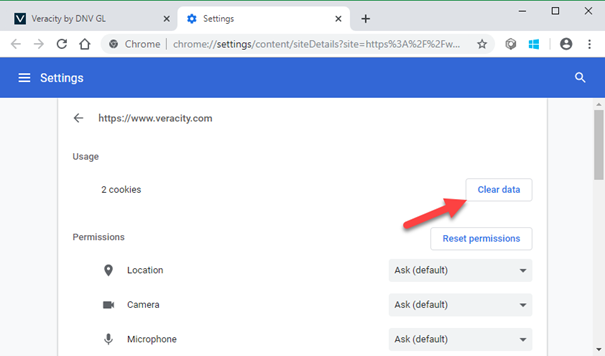A screenshot of the "Site Settings" page for the website "Veracity by DNV GL" is displayed in the Chrome browser. At the top, the browser tab reads "Settings." Below this, there is a distinctive blue navigation bar with the word "Settings" in white text on the left, accompanied by a white icon of three horizontal lines. The main section features a white box labeled with the URL "https://www.veracity.com" and a leftward pointing arrow.

Further down, details about the site’s data and permissions are presented. It shows "Usage: 2 cookies" and a "Clear data" button next to a red arrow pointing at it. The permissions are listed below, including options for "Location," "Camera," and "Microphone," all set to "Ask (default)" in gray boxes, each with a downward-pointing arrow for more options.

On the far right, there is a vertical scrollbar partially filled with gray at the top, indicating the user can scroll down for more settings information. Iconography is present to the left and right of these options, helping to visually categorize the settings.